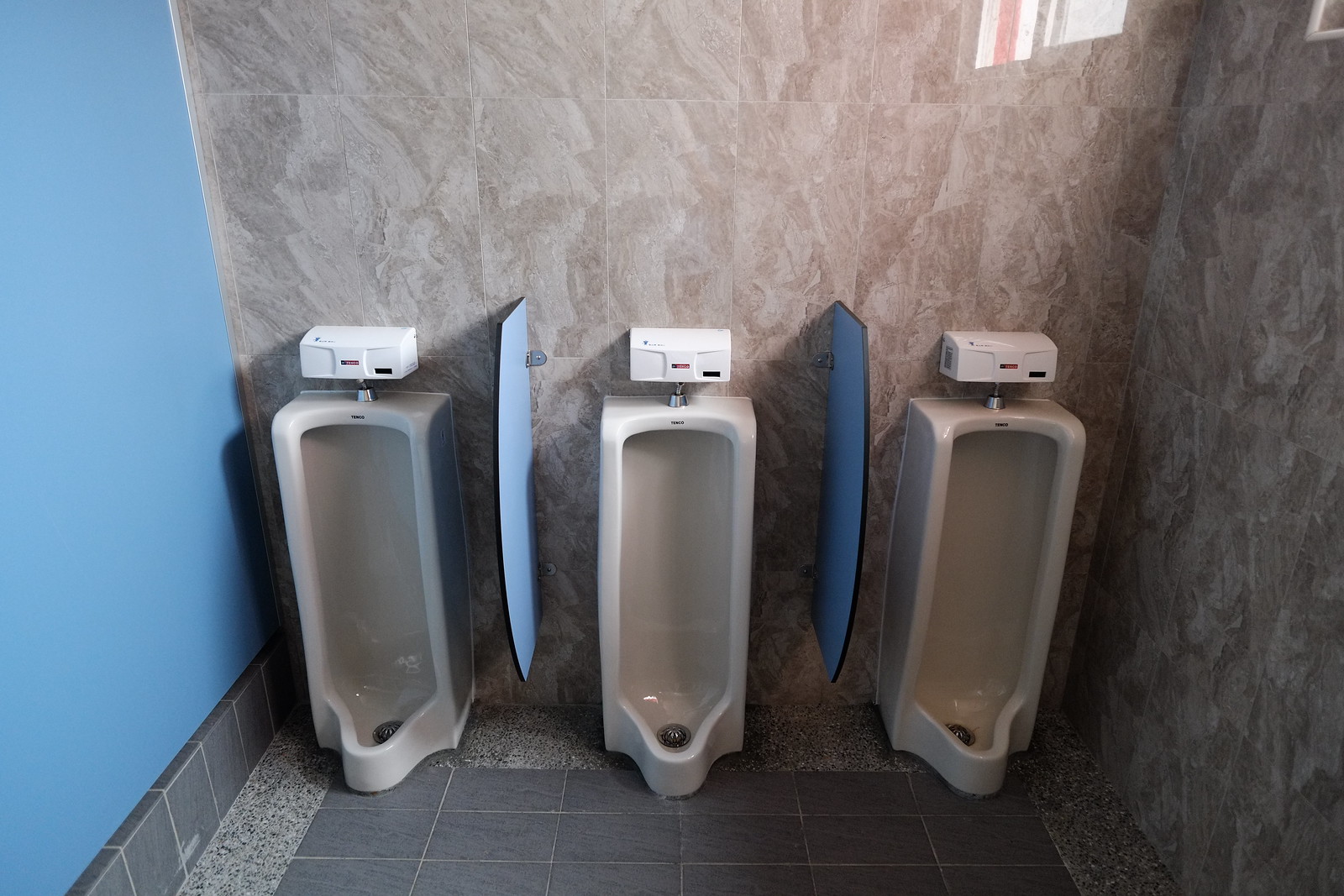The image is a detailed perspective of a men's bathroom featuring three white urinals. The urinals are positioned on a floor composed of a gray granite border with central dark gray textured granite tiles. Each urinal is equipped with a white automatic flushing box connected by a silver port. These urinals are separated by horizontally placed pale blue partitions. 

The left wall of the bathroom is painted blue, and the urinals are mounted against a wall tiled with large brownish marble panels. A gray baseboard tile, consistent with the floor tiles, runs along the bottom of this wall. On the right side of the image, another similarly tiled brownish marble wall can be seen. A window, though not visible in the image, casts sunlight onto the middle urinal, creating shadows that suggest the light is coming from the right side of the room. This creates a dynamic lighting effect, highlighting the central urinal more prominently than the other two. Overall, the bathroom appears clean and well-maintained.